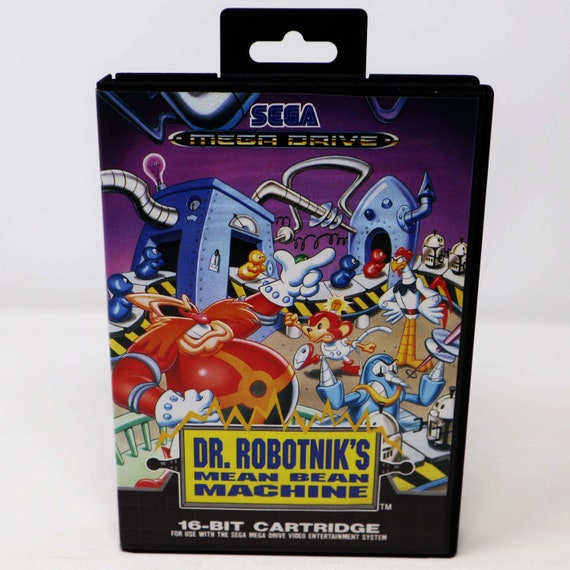This image features a Sega Mega Drive (also known as Sega Genesis) cartridge set against a plain white background. The cartridge, enclosed in a hard plastic case, has a hook at the top, designed for retail display on a metal rack. Dominating the front cover is an eccentric collection of cartoon characters, set against a backdrop that appears to depict a robot factory. Central to the image is Dr. Robotnik, a large, portly character with a conspicuous red outfit and an impressive brown mustache. Surrounding him are various quirky figures, including a small mouse in a white outfit, a conspicuous large chicken, and other mechanical elements indicative of a factory environment. The game's title, "Dr. Robotnik's Mean Bean Machine," is prominently displayed in blue font within a yellow rectangle near the bottom. Directly below this, a black banner with white text states, "16-bit cartridge for use with a Sega Mega Drive video entertainment system," emphasizing the compatibility and format of the game.